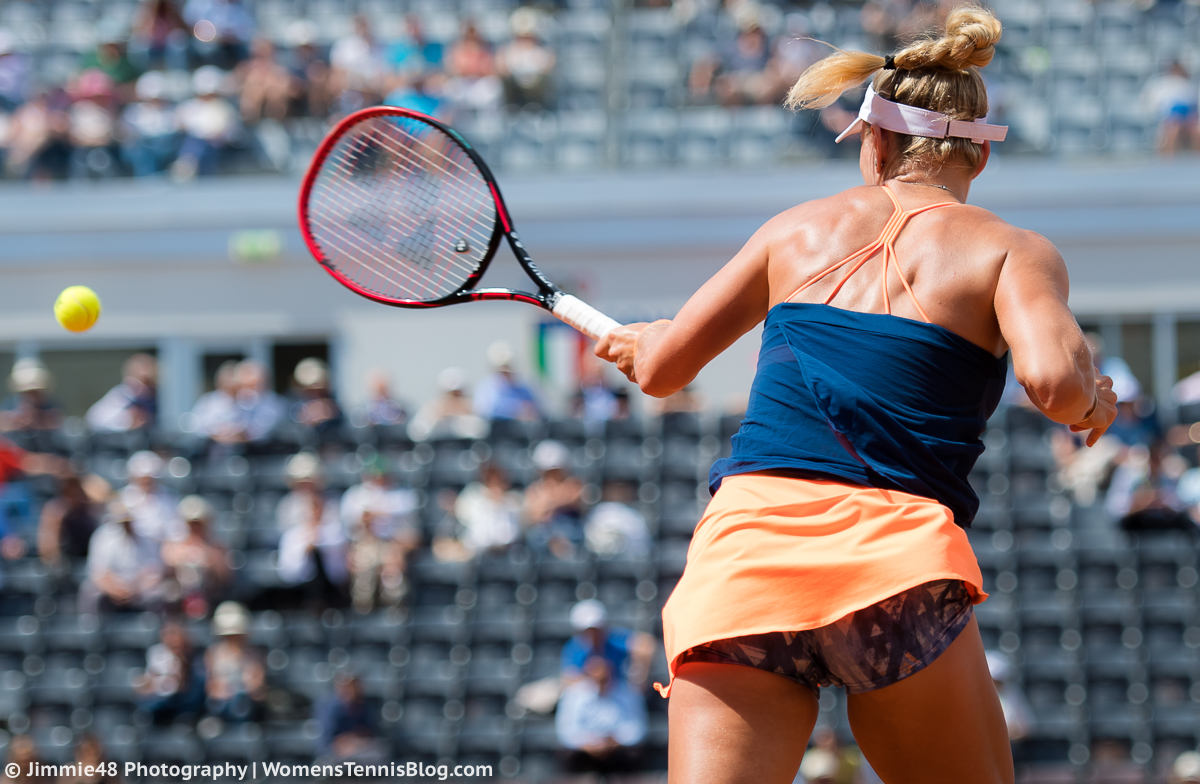This action-packed photograph captures a female tennis player, illuminated by bright sunlight under a clear blue sky, mid-play during a daytime outdoor match. She is positioned with her back to the camera, showcasing her turquoise green top, which features a unique design: four straps converge into a central point between her shoulder blades, and two additional straps extend over her shoulders. The player’s blonde hair is intricately braided and forms a ponytail that flutters up in motion. She dons a crisp white visor that secures her hair away from her face.

In her left hand, she wields a tennis racket with a white handle and predominantly red frame. The racket's strings are also red and interspersed with black geometric designs, including circles and triangles. The tennis ball, possibly just struck, is visible in mid-air on the left side of the image.

Her attire includes a pink skirt that has lifted due to her dynamic movement, revealing a pair of athletic pants underneath, which appear to be decorated with a subtle pattern of triangles. Her legs, visible from mid-thigh downward, exhibit the toned physique of an athlete.

The background reveals a sparsely populated stadium with blurred spectators, their presence only hinted at by groups scattered across the seating areas, making the player stand out as the clear focal point of the image. The stadium’s muted activity contrasts with the energy and precision of the tennis player’s performance, encapsulating a moment of intense athletic prowess.